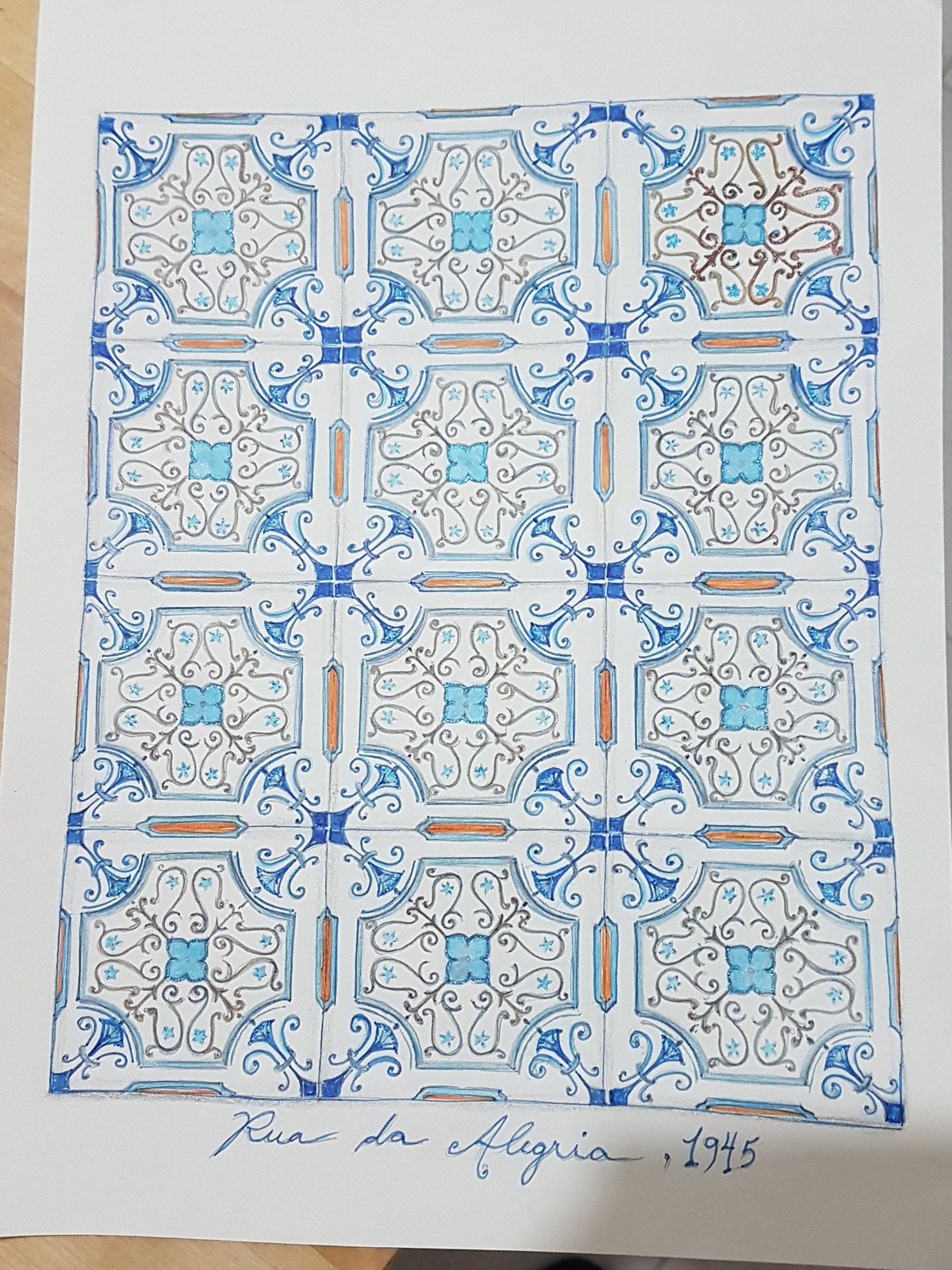The image captures a photograph of an art piece situated on a light brown table. The artwork, laid out on a white sheet of drawing paper, depicts an intricate tile pattern. This pattern consists of 12 tiles arranged in a grid of 3 horizontal and 4 vertical tiles. Each tile features a central design characterized by floral and intricate vine motifs, set against a white backdrop. The primary colors used in the design include light blue, dark blue, and orange, with additional accents of gold and brown.

At the corners of each tile, there are four circles with embedded embroideries resembling two interconnected C-shapes with curly Q ends. These C-shapes are joined by a centerpiece that appears metallic. Between the C-shapes, there are inward-facing fluke-like forms, akin to curved rectangles with pointed ends.

A prominent feature within each tile is a dark blue square containing a light blue flower-like shape. This central motif is adorned with glittering elements in the dark blue areas, a small bluish-gray circle at its heart, and curly Q embellishments in gold and brown hues. Interspersed among the curly Q's are small blue stars and flower-like patterns in brass and brown.

The artwork is signed at the bottom in cursive script, reading "Rua da Alegria, 1945". This detail suggests either the piece's title or a nod to a specific style and year, implying that the design might originate from this period. The signature and date are rendered in blue ink, adding a personal touch to the overall presentation.